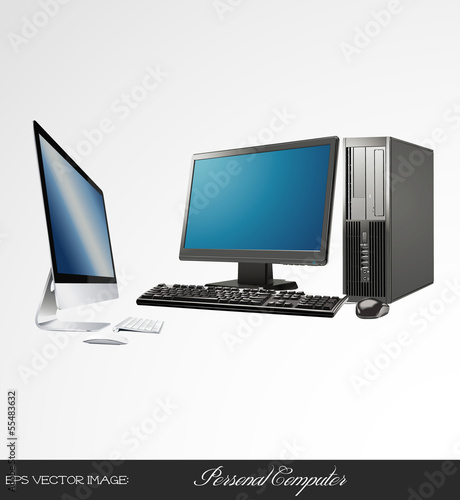The image showcases a meticulously arranged computer setup featuring both a traditional personal computer and a Mac. The background is a light gray to white gradient, prominently watermarked with "Adobe Stock" throughout. Centered in the image, a sleek, black-framed flat-screen monitor displays a gradient blue screen. Positioned in front of this monitor is a black keyboard with an adjacent black and gray mouse. To the right of this setup is a tall, gray computer tower with black vertical slots and a grille-like design at the bottom.

To the left, a thin, iMac-style, all-in-one computer with a black-bordered screen also displays a blue gradient image, intersected by a white diagonal line. The accompanying peripherals include a white Apple Magic Keyboard, angled with the left side facing the viewer, and a matching slim white Magic Mouse.

At the bottom of the image, a black rectangular strip runs across, featuring the text "EPS vector image" on the left and "personal computer" in elegant white cursive lettering in the center. The combination of equipment and the artistic gradient background creates a balanced, visually appealing composition ideal for stock imagery.